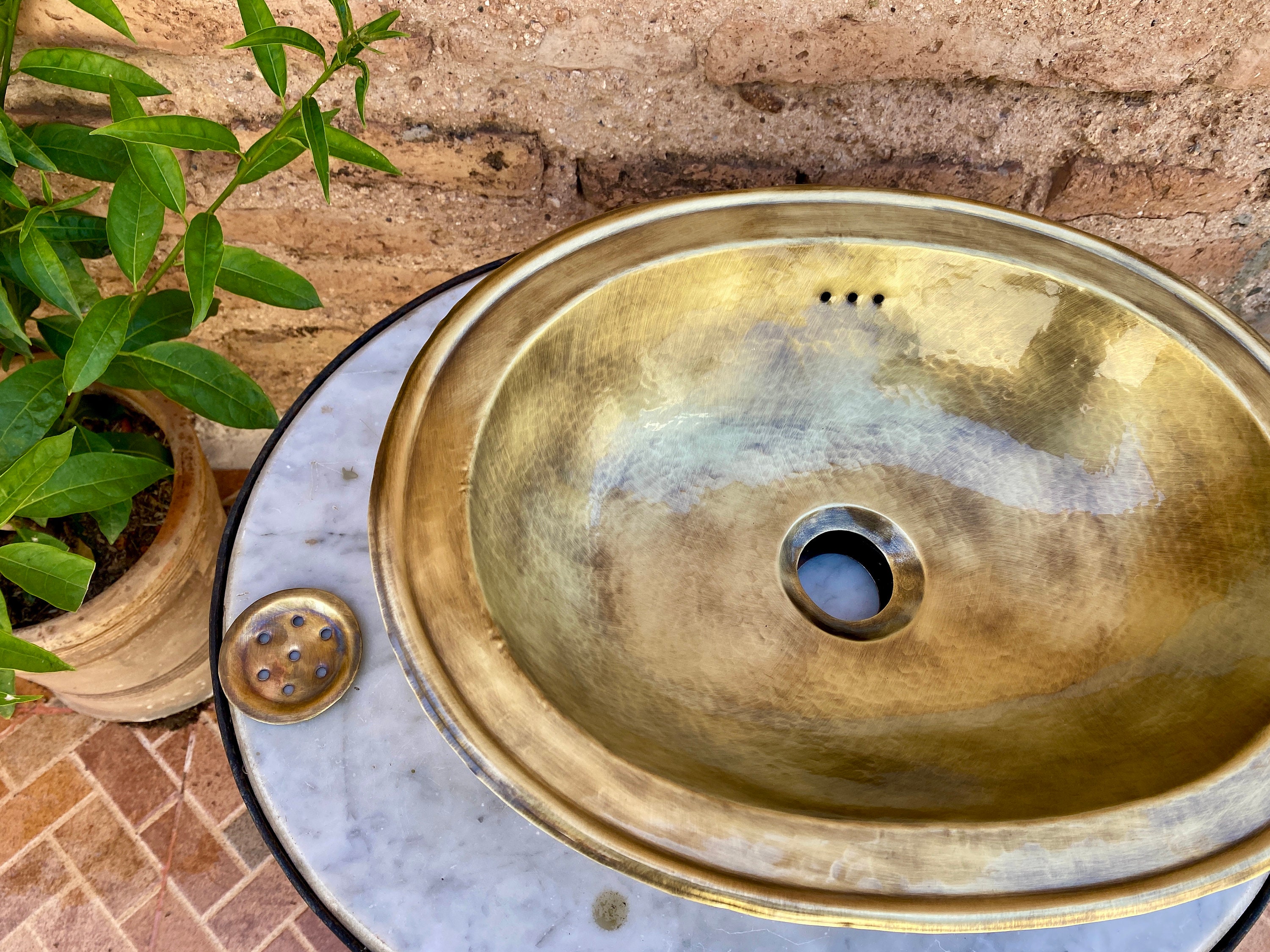This outdoor photograph, taken from above, captures a bright, sunny day. The ground is made up of interlocking bricks in various shades of brown and gray, forming a patio-like pattern. In the immediate foreground, there's the top of a circular patio-style table with a marble-colored surface and a black rim. Dominating the table is a large, shallow, brass sink bowl with a wide rim and a central hole, featuring a tarnished finish. Next to the sink bowl lies a small, circular brass object resembling a drain cap or ashtray, with six holes encircling one central hole. To the left of the table, there's a tan, barrel-like flowerpot containing a tall plant with long, green branches and leaves. This scene is set against a weathered brown brick wall with hints of tan-colored bricks inlaid, creating a rustic backdrop for the detailed patio arrangement.